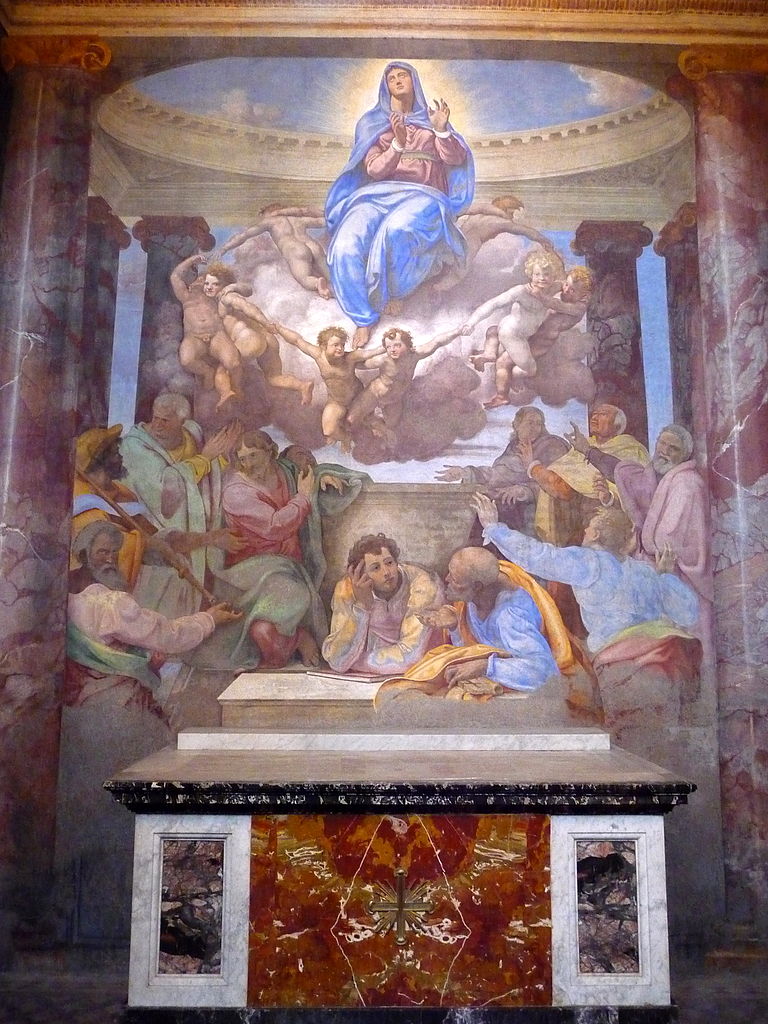This is an intricately detailed religious painting set in a historical chapel. At the very top, Mother Mary, dressed in a blue robe with a natural-colored bottom, sits on a cloud, a golden glow radiating behind her head. She is surrounded by angelic cherubs, some of whom appear more mature with features such as beards. The cherubs are depicted dancing and holding hands. Below Mary, a group of holy men in various robes, including blue and gold-and-yellow, stand and engage in discussions, with some looking up towards her. The chapel interior features marble pillars, with some individuals in period attire sitting and reading books. The background sky is a serene blue dotted with puffy clouds, and at the very base of the painting, there's a plinth adorned with an indistinct religious symbol.